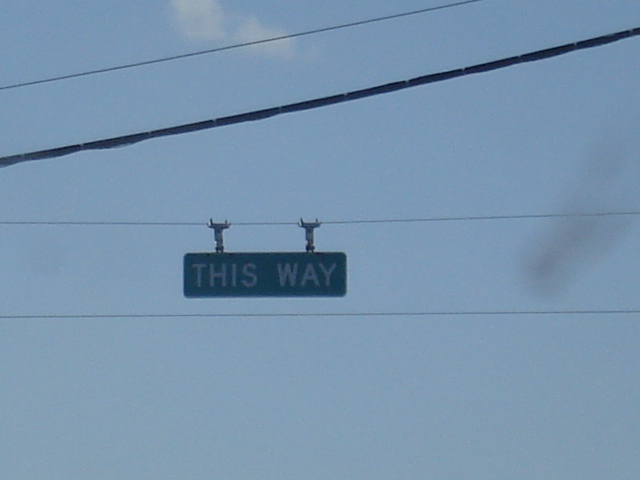The image features a rectangular street sign that prominently displays the text "THIS WAY" in bright white, capitalized, impact font against a greenish background. The sign is suspended by two thin metal clamps, one positioned above the word "THIS" and one above the word "WAY," which are fastened to what appears to be a telephone wire. The sign is centered in the image, hanging among a series of wires. In addition to the wire holding the sign, there is a thicker black wire extending diagonally from the bottom left to the top right of the image, as well as another thin wire running parallel above it.
 
The background of the image consists of a mostly clear, pretty blue sky with varying descriptions of clouds. There is one small, white cloud near the top left and another faint, grayish cloud in the middle right side of the image. Additionally, there is a very blurred image of what might be a tree branch in the scene, adding a subtle, fuzzy element to the photo.